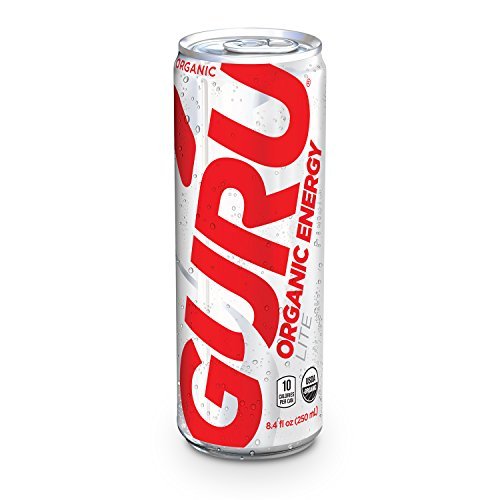This image features a tall, slender canned drink, approximately seven inches in height and three inches in width. The can predominantly has a silver color with distinguished textual and label elements. From top to bottom, bold red uppercase text spells out "GURU," with "Organic Energy" in smaller red text directly below it. Further down, "LITE" is displayed in white or silver text. Below these textual elements, there are two labels within circles. The first circular label reads "10 calories per cup" while the second comprises "USDA Organic" with “Organic” repeated in the lower half of the circle. Additionally, the top right features the word "Organic" in red text. Towards the bottom of the can, the capacity is marked as "8.4 fluid ounces (260 milliliters)" in red text. The can is topped with a silver flip-tab for opening, which contrasts against its silver border.